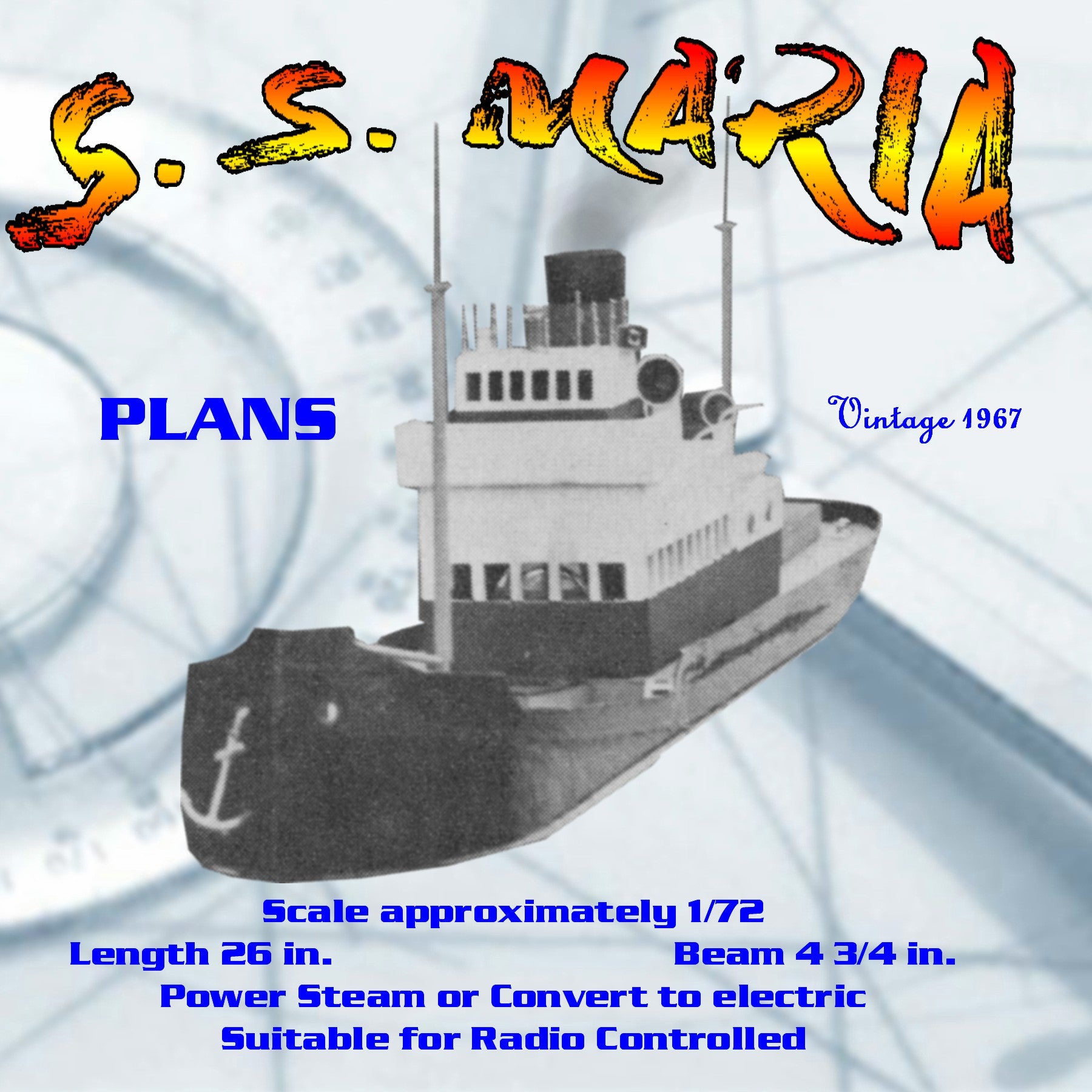The poster features an old inset photograph of a steam-powered ship named the S.S. Maria. The ship is depicted in a black and white cutout, with a prominently highlighted anchor at its front due to its lighter color against the dark hull. The vessel includes two large poles, known as masts, positioned at the front and back. Centrally located, the cabin appears to be at least two stories tall with multiple windows around the sides and front. Above the image, the text "S.S. Maria" stands out in yellow and orange letters. Below this, blue text reads "Plans, Vintage 1967." Additional blue text at the bottom specifies the ship's scale as approximately 1/72, with a length of 26 inches and a beam of 4¾ inches. It notes the ship can be powered by steam or converted to electric, and is suitable for radio control. The image as a whole is reminiscent of a vintage blueprint or model kit advertisement.